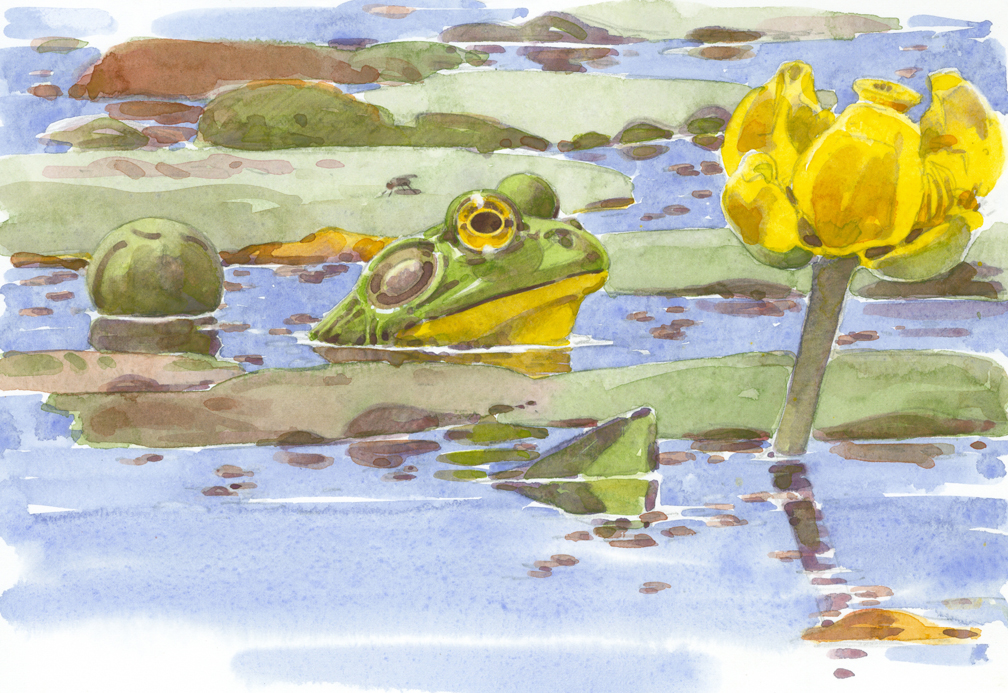This detailed, landscape-oriented watercolor painting captures the serene scene of a bullfrog resting in calm, light blue water with white hues. The bullfrog, positioned at the center of the composition and facing to the right, showcases a vibrant palette with its predominantly green body accented with darker green spots. Its distinctive yellow throat and bright yellow eyes draw attention, while its brown earpieces contrast subtly. Surrounding the frog, lily pads float scattered on the water's surface, complemented by a prominent yellow lily flower emerging on the right. Further enhancing the aquatic setting, hints of vegetation and brownish debris are delicately sprinkled, adding texture and depth to the tranquil environment.